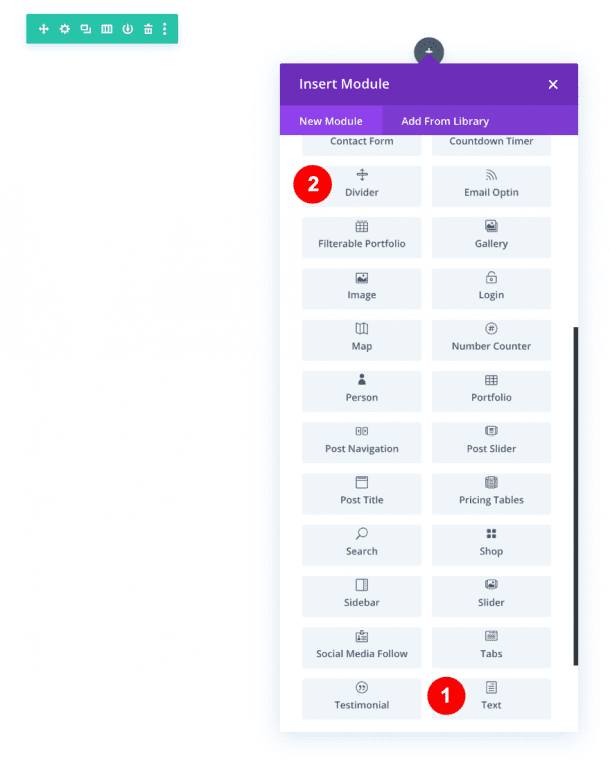This detailed screenshot showcases a control panel from a website builder interface. The upper portion prominently displays an "Insert Module" section featuring two tabs: "New Module" and "Add from Library." The current view highlights the "New Module" tab, which is open to display various module options. Notably, two areas within this screenshot are marked with numbers inside small red circles. The "1" is positioned next to the "Text" module option, while the "2" is adjacent to the "Divider" module option.

In the upper left corner of the screenshot, there is a compact control panel housed within a green square or rectangle. This panel includes several navigation and functional icons, such as a gear (settings) icon and a download icon, amongst others.

Overall, the interface appears to be a robust, user-friendly website builder allowing users to customize their webpages by inserting and arranging various modules like text and dividers. The presence of search and sidebar options further implies extensive customization capabilities, facilitating the construction and organization of comprehensive web content.